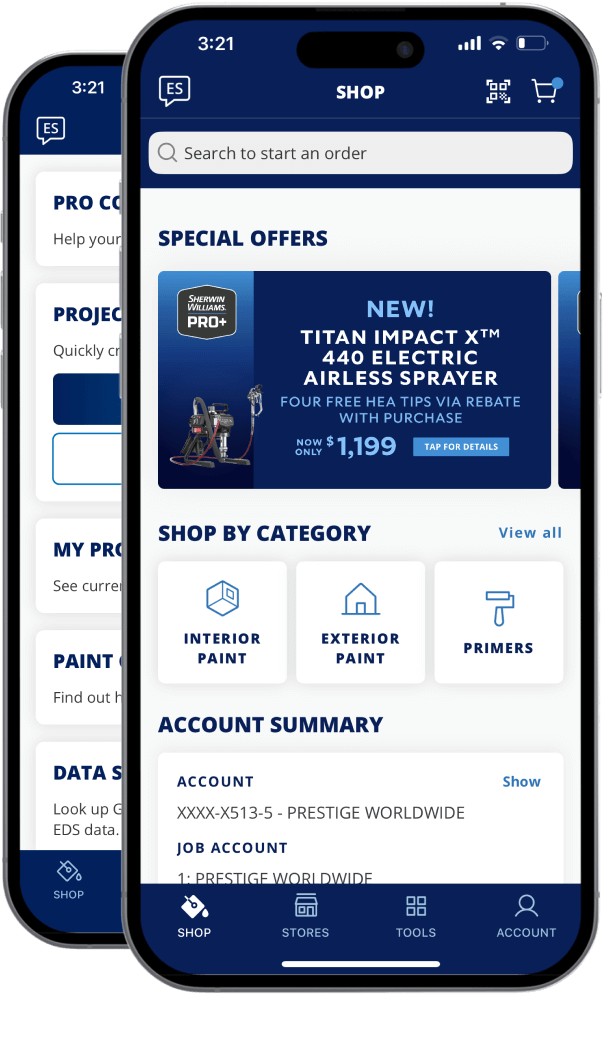The image depicts two gray smartphones displaying a home improvement app or website interface against blue backgrounds. 

**Front Phone:**
- **Top Section:** Displays "3:21" on a blue status bar alongside a small white square with "ES" inside. Below, there's a navigation bar featuring icons for 'Shop' and a shopping cart symbol with a blue dot notification indicator.
- **Search and Offer Section:** Features a prominent white search box, followed by a large white banner titled "Special Offers." Beneath this is a substantial blue box displaying promotional content for the "New Titan Impact X 440 Electric Airless Sprayer," highlighting a free HEA Tips via rebate offer and a price of $1,199.
- **Categories Section:** Showcases a blue button labeled "Top Offers." Below, there’s another blue box with the label "Shop by Category - View All." Inside this box, there are three white sub-boxes categorizing products into "Interior Paint," "Exterior Paint," and "Primers."
- **Account Summary:** A white box details the account summary, showing "Account" and a "Show" button on the right, along with some numbers and the text "Prestige Worldwide Job Account."
- **Bottom Section:** Features a dark blue navigation bar with icons for 'Shop,' 'Stores,' 'Tools,' and 'Account.'

**Partial View of the Second Phone:**
- **Top Section:** Also displays "3:21" with "ES" inside a white square and similar application layout elements.
- **Content Section:** Displays text mentioning "Pro something" and "Help your project," accompanied by a blue and a white box with "My Project Paint and Data."
- **Navigation Bar:** Similar to the front phone, it includes icons for 'Shop' and other essential features at the bottom.

This detailed depiction covers various UI elements and sections catered to shopping, offers, categories, and account management on a home improvement app or website interface.